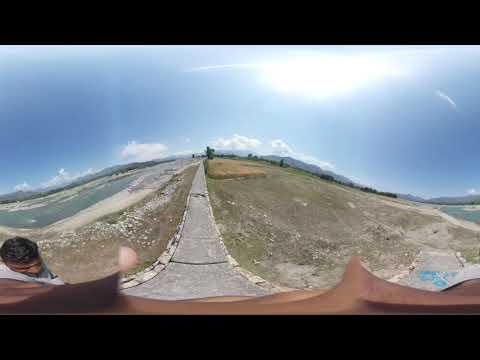The image is a color photograph captured likely with a GoPro, characterized by a fish-eye lens effect that distorts the front end. It portrays a cement trail that extends from the bottom center of the image, curving towards the left, creating an illusion of descending and then ascending like a massive hill. This distortion is enhanced by a panoramic filter and an Inception-style grid filter, seamlessly merging three photographic perspectives into one composite view. On the left and right edges of the image, there appear to be curved shorelines, possibly of a lake or ocean, blending into the open land space. The land is beige and green, with different shades of brown, suggesting a natural landscape. In the center, where the trail ascends the hill, the landscape continues upward, culminating in a few green trees on the horizon. A partly cloudy blue sky with the sun beaming from the top center-right of the image forms the backdrop. At the bottom left, a Middle Eastern man with brown skin and black hair, cropped and looking down, appears distorted due to the fish-eye effect. Additional indistinguishable light blue features are spread out horizontally at the very bottom, further contributing to the warped perspective.